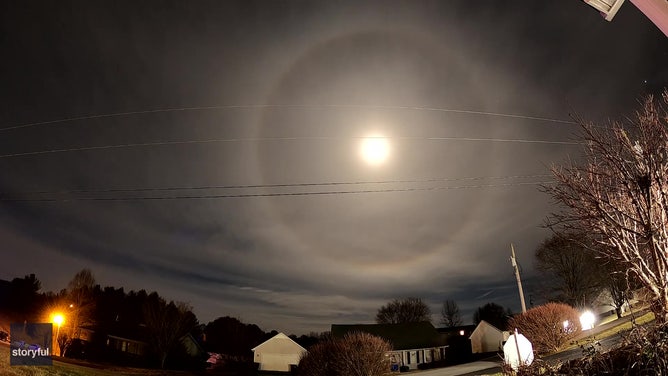This nighttime photograph vividly captures a quiet neighborhood under a striking night sky. Dominating the center of the image is a bright, full moon encircled by a luminous halo, casting a surreal glow on the surroundings and piercing through the dark gray clouds. The silhouette of power lines crisscrosses the moon, accentuating its brilliance. In the bottom left corner, a watermark reads "Storyful." The scene includes several single-family houses with dark roofs, some with driveways and garages, scattered across the neighborhood street. A few outdoor lights are turned on, adding a subtle warmth to the otherwise dark scene. Bare trees and bushes, indicative of autumn or winter, frame the houses and hint at the season. The composition also includes the back of a stop sign and a streetlight, with darker, more distant trees completing the backdrop. The overall focus remains on the glowing moon and its ethereal halo, which illuminate the tranquil neighborhood below.